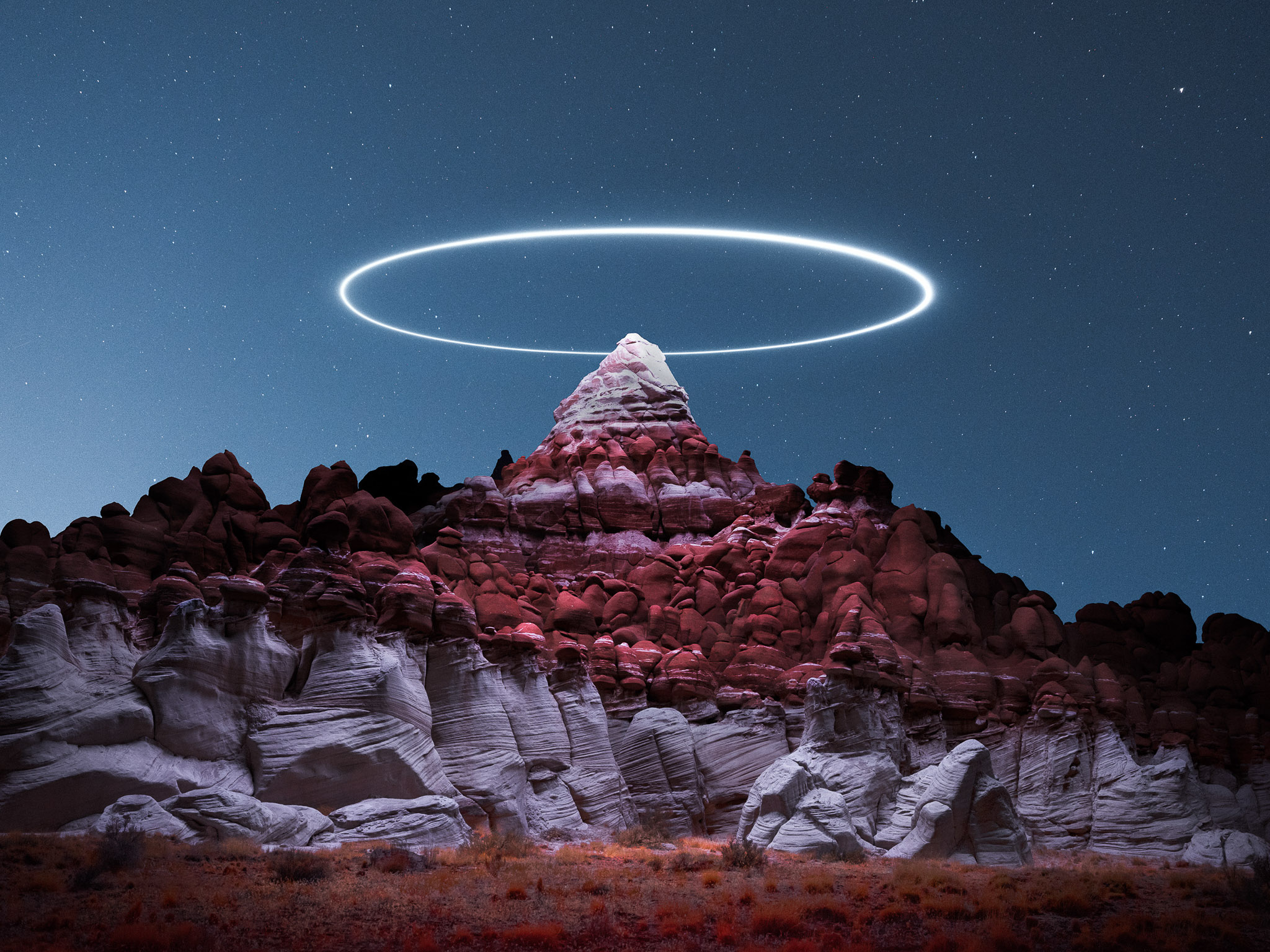This detailed nature photograph captures a mesmerizing desert scene dominated by a multi-colored rocky hillside. The base of the hill features smooth, white rocks interspersed with sparse tufts of red and orange grass. As the hill rises, the rocks transition through an array of colors: from coral pink and deep purple to vibrant red. Higher up, particularly towards the peak, the rocks adopt a darker red hue before tapering off into a near-white, pointed peak. A striking feature of the landscape is the ethereal white halo of light hovering just above the peak, casting an artificial illumination over the scene. The background sky is a dark, deep blue, filled with thousands of stars and a few clouds, enhancing the surreal and otherworldly atmosphere of this nighttime scene.